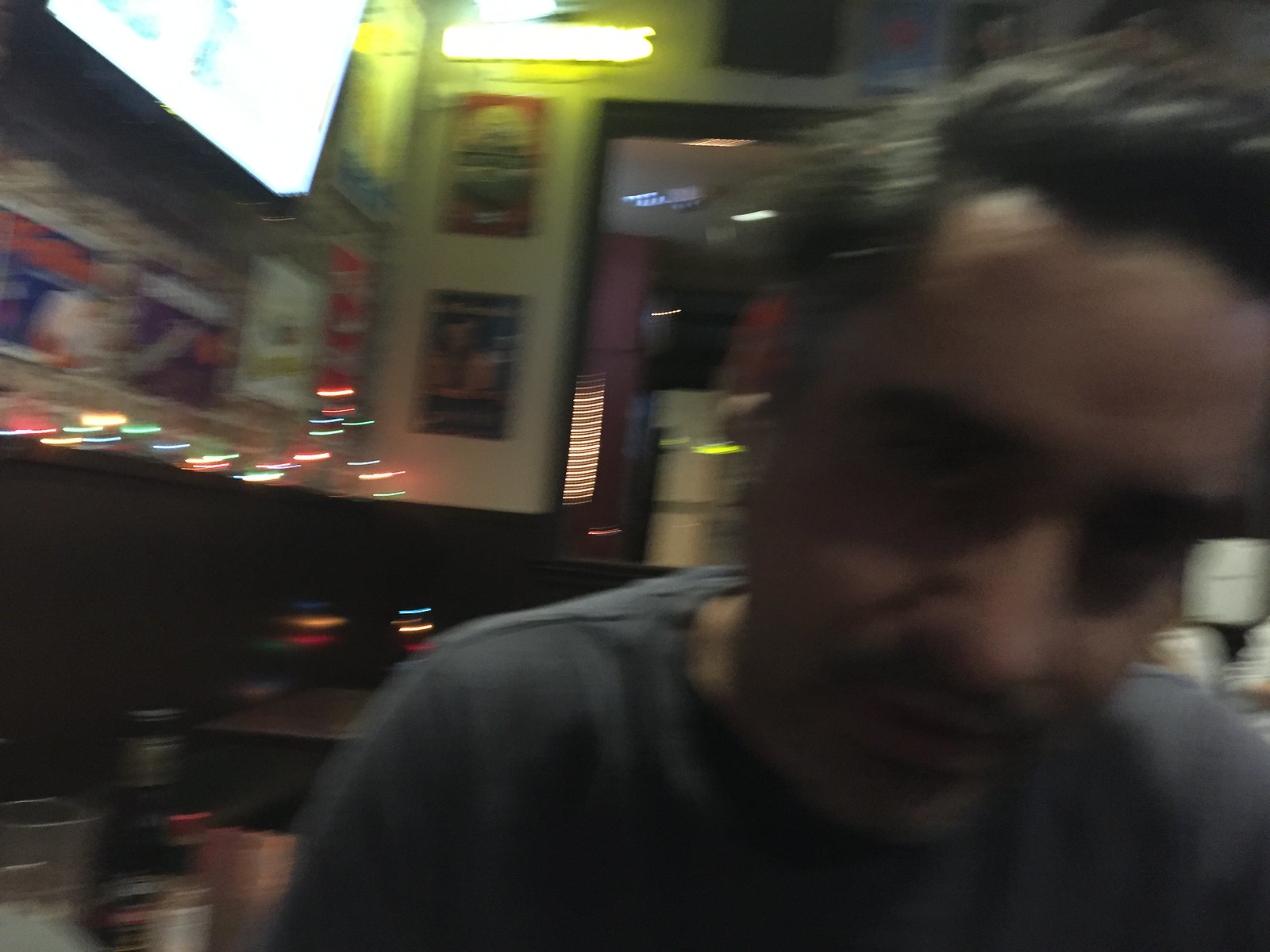The image features a close-up, albeit very blurry, of a man sitting in what seems to be a restaurant. The shot captures his figure from around the mid-upper arm up, allowing a detailed view of his head and shoulders. He has a light tan complexion and thick, black hair neatly parted to the side. His eyes are obscured by shadows, but his prominent nose, black mustache, and mouth are visible. The man is dressed in a dusty bluish-gray t-shirt and is leaning slightly forward with his head tilted to one side.

In the background, there's a table to his side holding a beer bottle and an empty glass. Further behind, there's an empty square wooden table. The brightly lit wall behind him is adorned with numerous posters and features a large screen TV that is turned on, creating a lively ambiance typical of a bustling eatery.